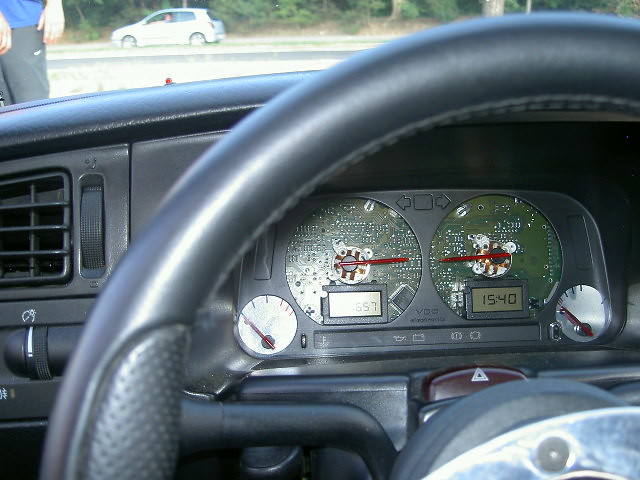This is a color photograph taken from inside a car, offering a close-up view through the top of the steering wheel, focusing on the dashboard. The dashboard appears incomplete, as some covers are missing, revealing the exposed electrical components where the gas gauge would typically reside. Visible on the dashboard are the numbers "1540" and "1657." Additional details include the windshield wiper control and the emergency button. Outside the car, two individuals are standing near the front of the vehicle. One person is dressed in a blue shirt and black pants, and their hands are visible. In the background, a small silver or white two-door car with its window down is present. The car's interior is entirely black, and the proximity of the photo gives the impression of being almost pressed against the steering wheel. The make and model of the car are indeterminable due to the close-up nature of the shot and the unusual, uncovered state of the dashboard.